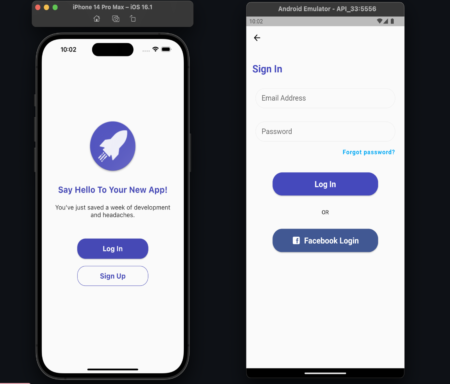Here's a detailed, cleaned-up caption for the image described:

---
The image features a black background. In the top left corner, there is a gray rectangular box with three colored circles, arranged horizontally from left to right: red, yellow, and green. This box contains some text that is too small and blurry to read. Below the box, a smartphone screen is displayed showing the time as 10:02, a full battery icon, and a strong Wi-Fi signal. 

The main part of the screen has a white background with a central blue circle containing a white rocket ship icon. Below the icon, blue text reads, "Say hello to your new app," followed by black text stating, "You just saved a week of development and headaches."

There are two buttons beneath this text: a blue button with white text that says "Login" and a white button with blue text that says "Sign Up."

On the right side of the image, another section with a white background shows an arrow pointing to the left with blue text that says "Sign in." Below this, there are two text boxes labeled "Email address" and "Password," respectively. A blue hyperlink that reads "Forgot password" is present below the password text box. Another blue button underneath this hyperlink says "Login." Below the button, the word "or" is displayed, followed by a darker blue button that says "Facebook Login" in white text.

---